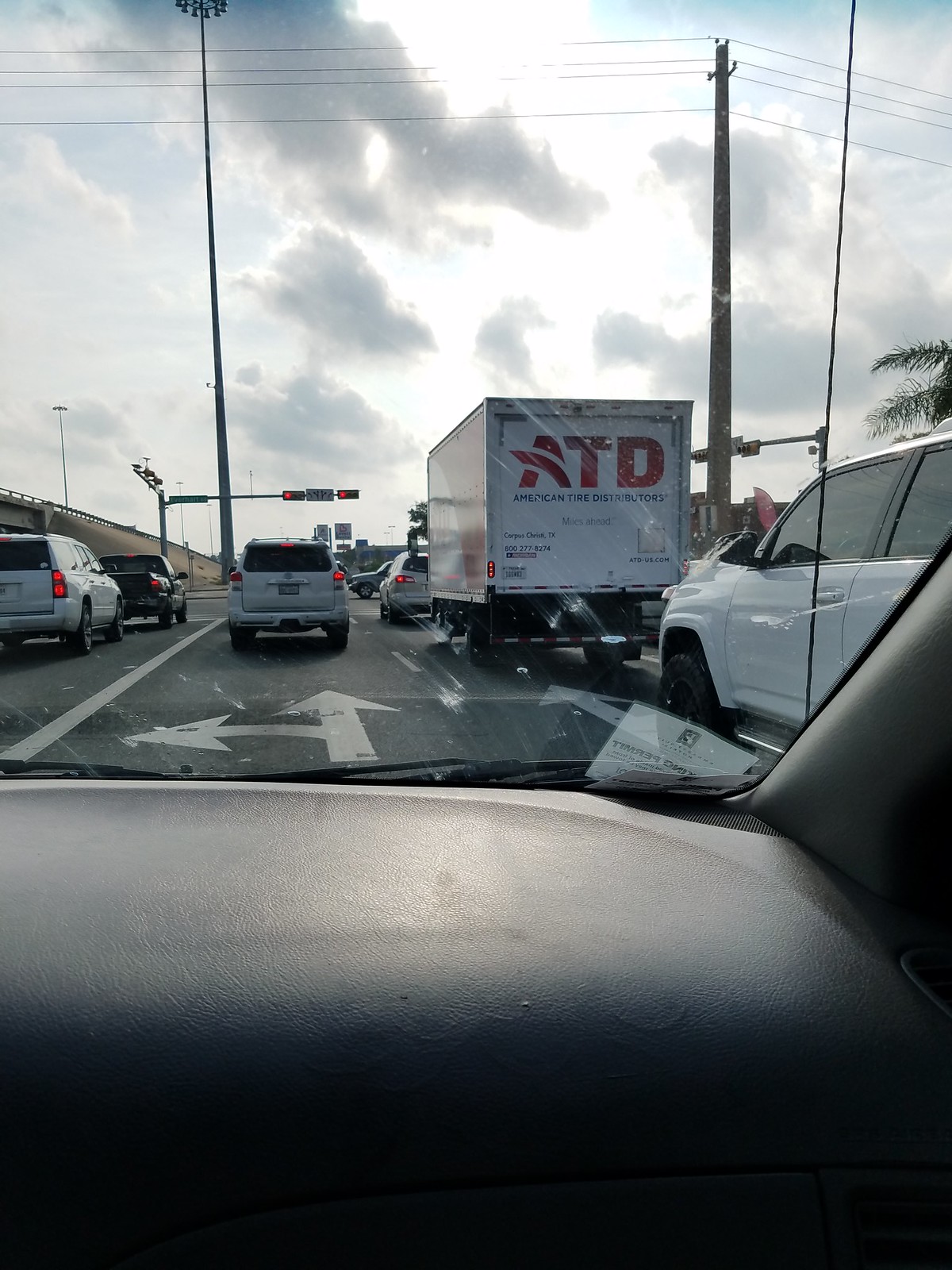The image captures a scene from inside a car, taken through the front windshield. The view shows traffic ahead and to the side of the vehicle. A small white card with unreadable text is also present on the windshield, and there are noticeable wiper marks. Directly in front, there is a white truck with "ATD" written on it, while another smaller truck in a different lane is not white. The car's dashboard, visible in the foreground, is black. The sky is heavily overcast with numerous clouds, indicating a very cloudy day. In the background, palm trees are visible, suggesting the location is in the southern region. The lane the car is in allows for both straight and left-turn movements.